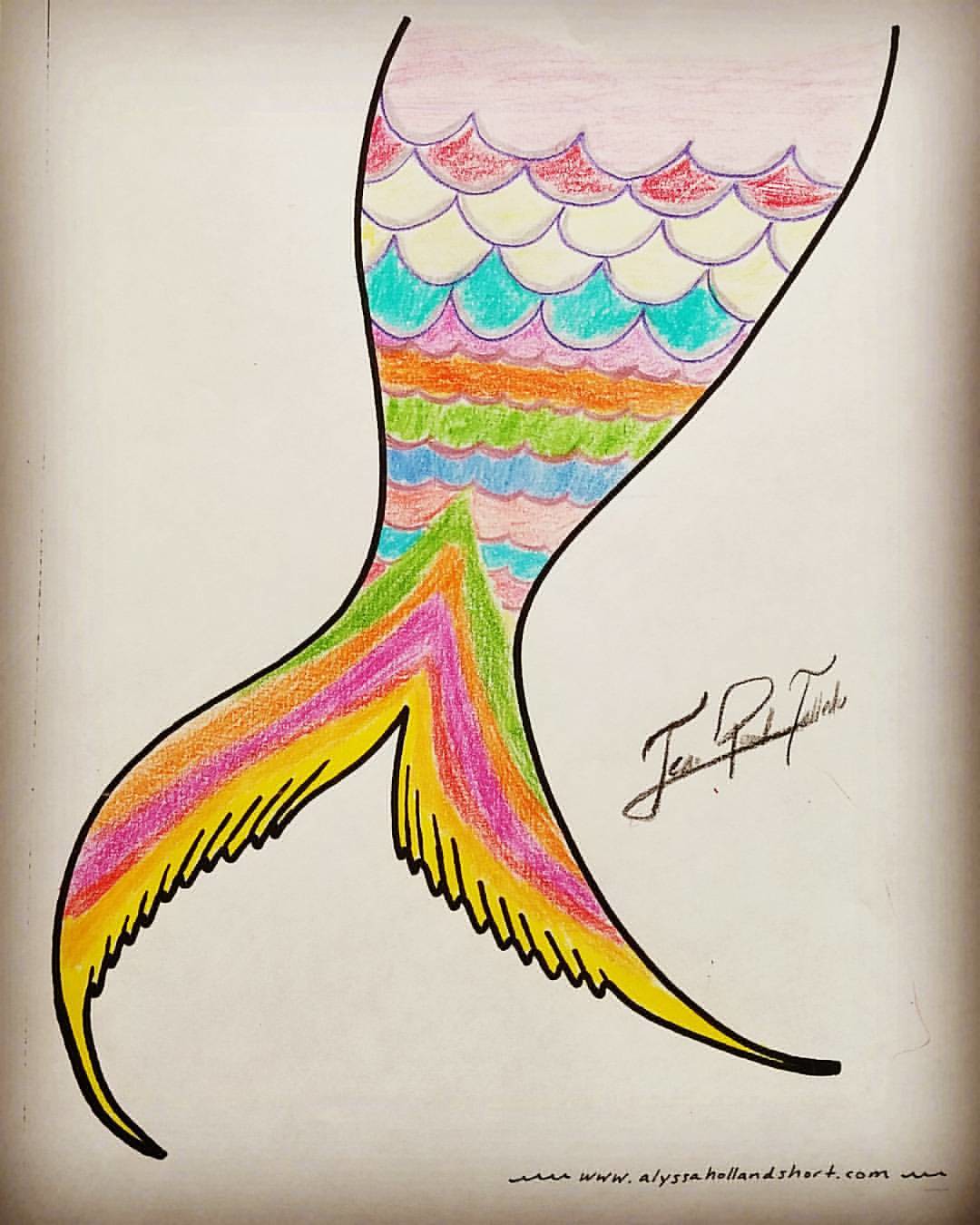The image showcases a meticulously detailed sketch of a fish's body outlined with smooth, flowing curves. At the bottom of the image, you will notice two fins. These fins have an intricate color gradient starting from the edges with yellow, transitioning to pink, orange, and green. Where the fins intersect with the fish's body, there is an elaborate pattern of horizontal lines in shades of purple, blue, pink, blue, green, orange, blue again, purple, blue once more, and finally white. The fish's main body is left a pristine white. In the bottom right corner of the image, there is a series of small black text, indicating a website. Additionally, a black cursive autograph graces the right side of the image. The background of the sketch is a subtle gray, lending a simple yet elegant backdrop to the vibrant colors and intricate details of the fish's design.